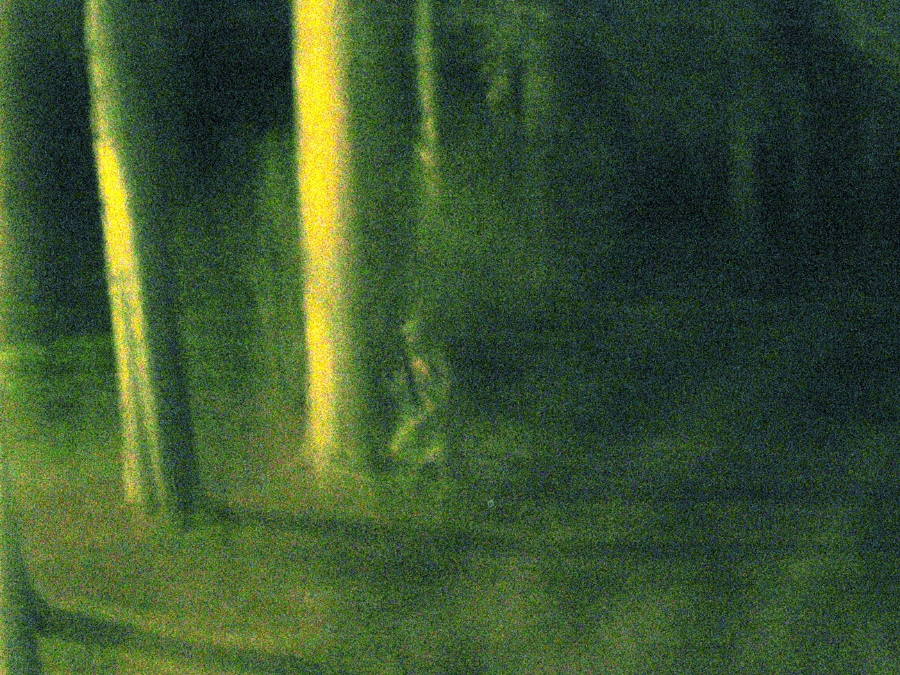The image is a night vision photograph, capturing a forest scene with varying green and yellow shades. It is quite blurry and fuzzy, adding a mysterious quality to the scene. In the foreground, large trees dominate, with additional trees visible in the background. A clearing is noticeable through the clustered trees. In the middle of the picture, a silhouette of a soldier, or possibly a person, is kneeling behind one of the largest trees, seemingly taking cover. The person appears to be holding a dark object, possibly a long gun. On the left-hand side of the picture, the tallest trees stand, with some foliage visible, though the color saturation makes it difficult to distinguish individual trees. The background is pitch black, adding to the eerie atmosphere. Light and dark shades of green and some blue are mixed throughout, particularly on the trees and the ground cover, giving the entire image a shaded and somewhat surreal appearance.